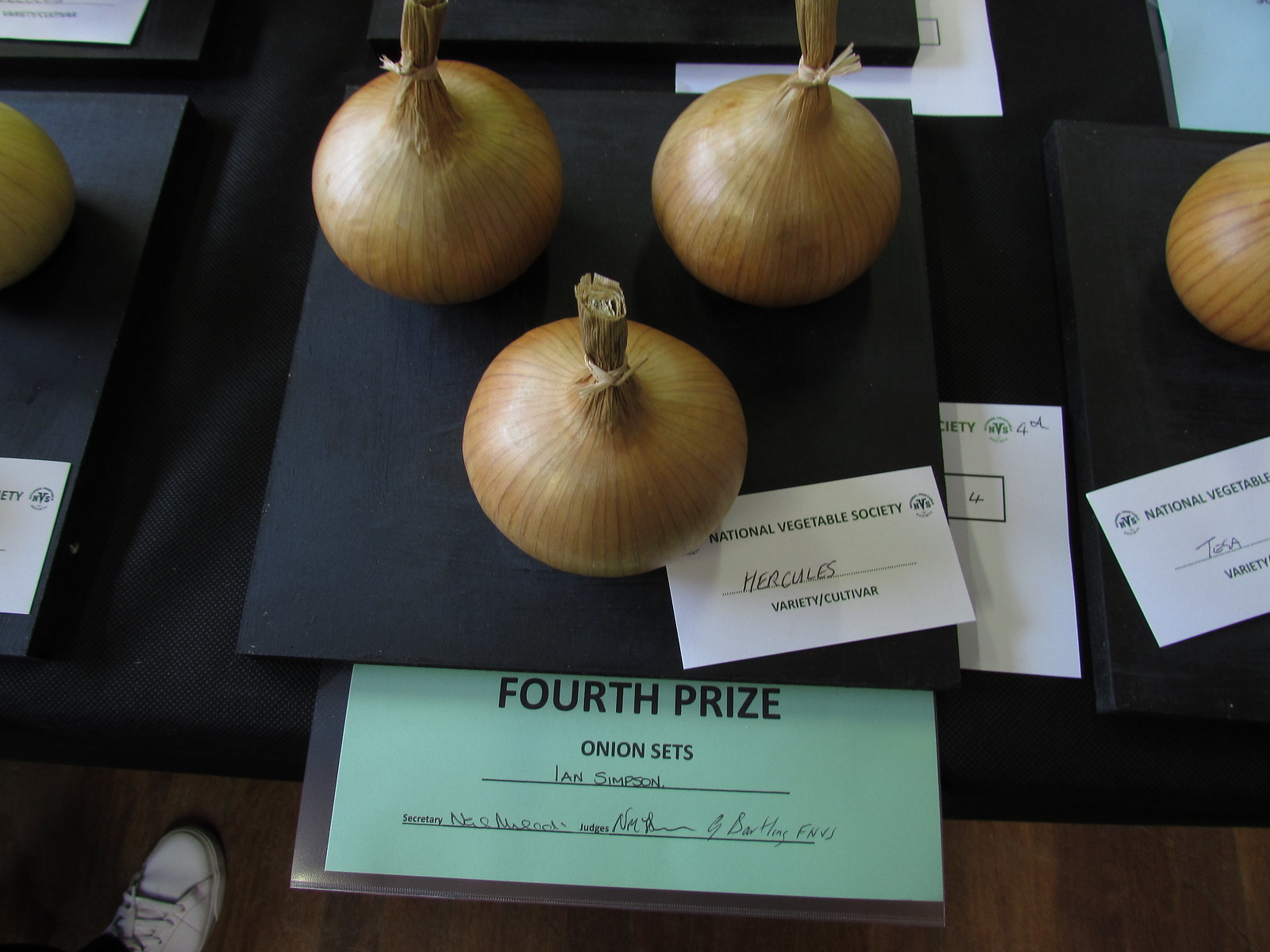The image prominently features three light brown yellow onions standing upright on a black square platform at the center. Each onion, with its brown wrapping intact, has its roots sticking upwards. Beneath this platform, a light green tag indicates "Fourth Prize Onion Sets" with the name "Ian Simpson" written on it, implying a competitive context, possibly a vegetable show. Directly below the onions, a white card reads "National Vegetable Society Hercules Variety/Cultivar." The background is predominantly black, highlighting the subject. To the left and right, partially visible, are additional onions on similar black platforms, accompanied by small white cards, suggesting other entries in the competition. At the bottom of the image, the tip of a white shoe peeks through, likely belonging to the photographer. The scene is well-lit with interior lighting.